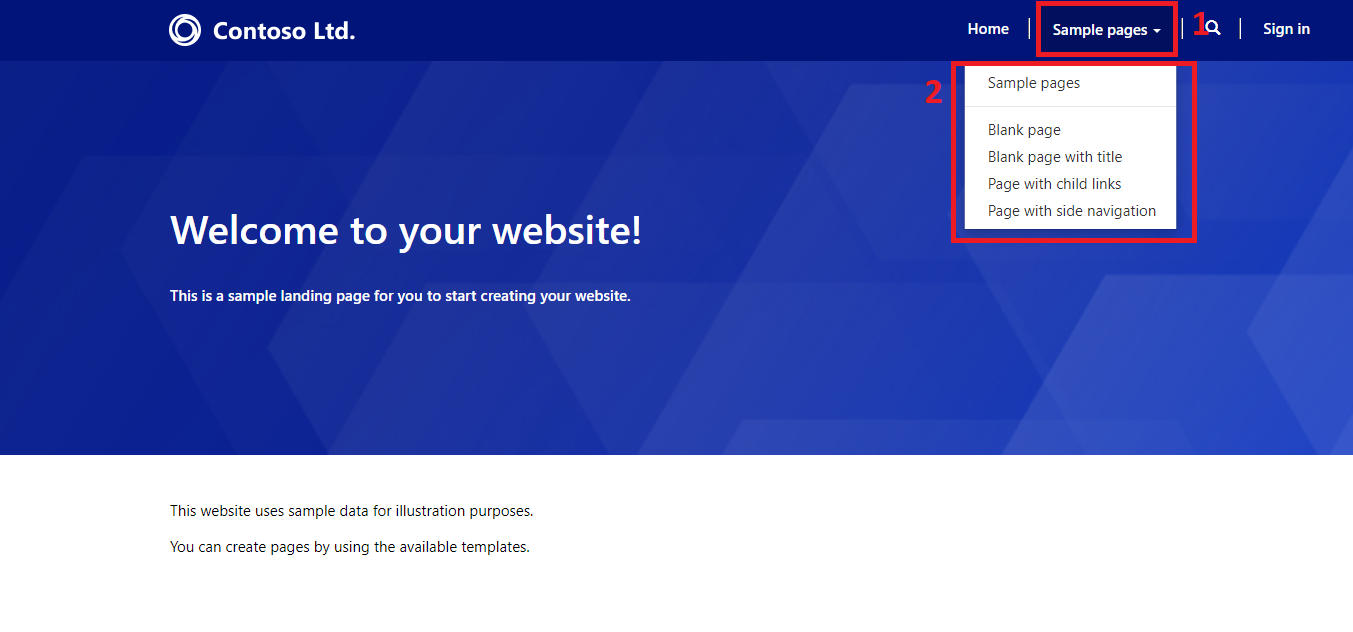This image showcases a professional website belonging to Contoso LTD. The top section of the website features a dark blue header. On the left side of the header, there is a circular icon or symbol representing Contoso LTD. To the right, the header includes navigation options such as “Home,” followed by a white separator line.

A red-outlined box appears next, with a blue interior, containing the text "Sample Patients" accompanied by a drop-down menu. Within this menu, highlighted by the red border, several options are listed: "Sample Pages," "Blank Pages," "Blank Pages with Title," "Page with Child Links," and "Page with Side Navigation."

Adjacent to the drop-down menu, on the far right, there is a number “1” marked in red. Additionally, a number “2” appears in red on the left-hand side of the drop-down.

The header also includes a magnifying glass icon for search functionality and a sign-in option labeled "Sign In."

The main body of the website has a light blue background with a subtle, faded triangle design. Prominently displayed at the center is a welcome message, "Welcome to Your Website," followed by introductory information about the site.